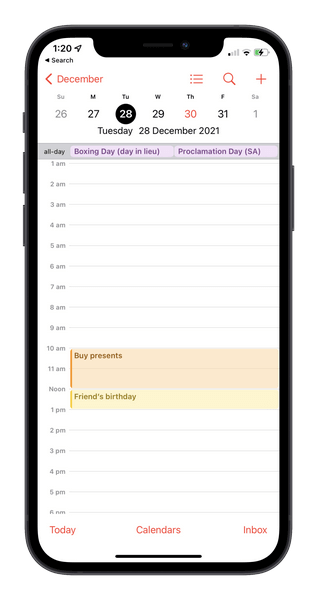This image features a close-up view of the Calendar app displayed on a black-framed iPhone. The sleek black device prominently showcases its signature design elements: the power button is located on the right side of the phone, while the left side houses the ringer switch at the top and the volume buttons just below it. 

The screen of the iPhone Calendar app is primarily white with subtle light gray lines demarcating the days and weeks. At the top of the screen, the month "December" is highlighted in red next to a back arrow, a list view button, and search and add icons positioned in the upper right corner.

On December 28th, which appears prominently in the calendar view, several events are scheduled. An all-day event labeled "Boxing Day, Proclamation Day" is shown in blue. Additionally, from 10 a.m. to noon, there is an event marked as "Buy presents," followed by "Friend's Birthday" scheduled from noon to 1 p.m. The detailed view provides an organized snapshot of the user's plans and important dates for the end of the month.